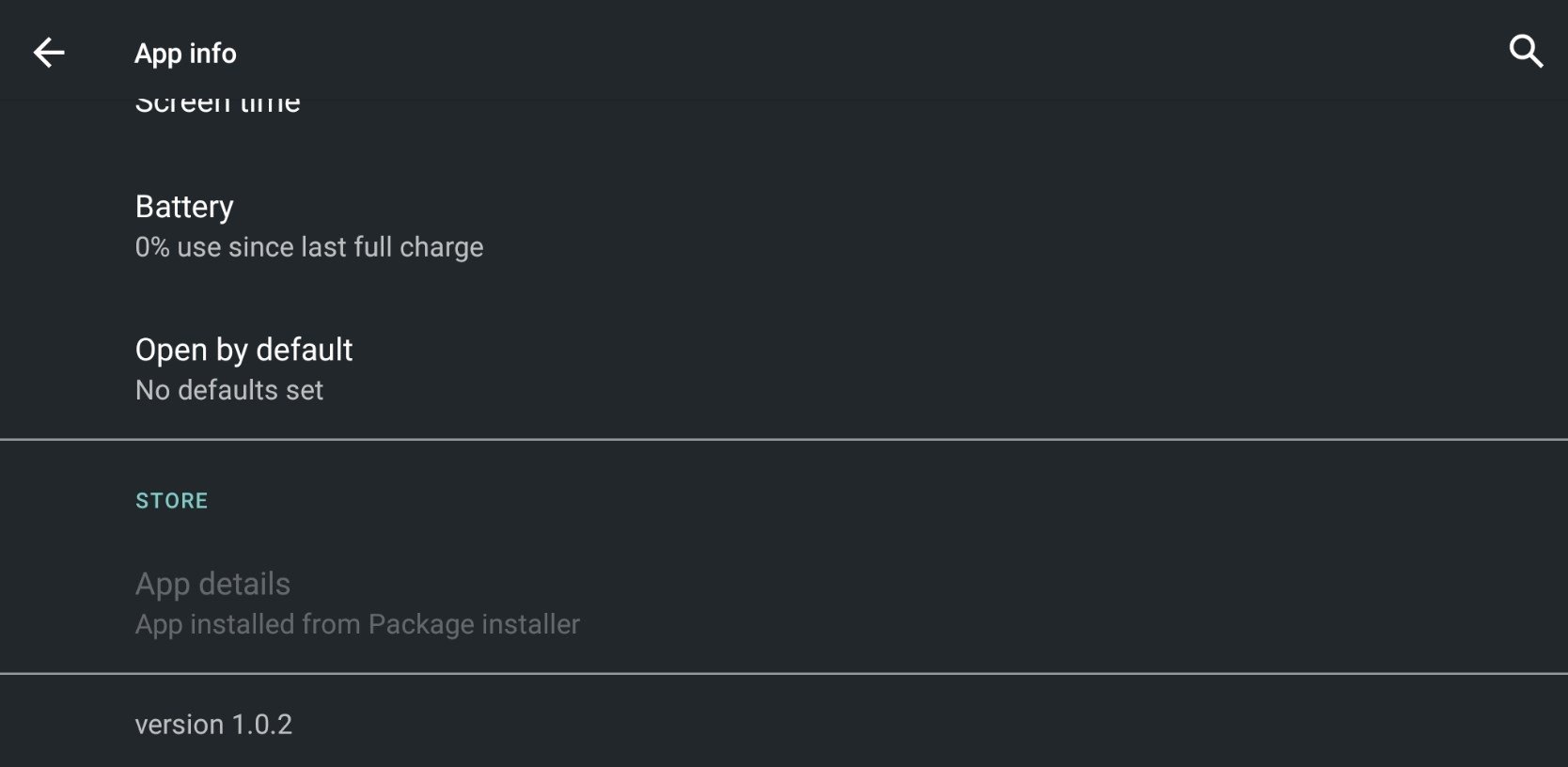A detailed screenshot of a technology interface or website is presented, featuring a predominantly black or very dark gray background. The interface includes white text, contrasting sharply with the background for readability.

In the top left corner, there is a left-pointing arrow, suggesting the option to navigate back. Adjacent to this, the header displays the words "App info." On the far top right, a search icon is positioned, providing a tool for finding specific information.

The main content of the screenshot is divided into segmented sections by two horizontal lines. The top section contains the following labels and information in white text:

- "Screen time"
- "Battery: 0% use since last full charge"
- "Open by default: No default set"

Below this section, there is a clickable item in blue labeled "Store." Underneath, in gray text, it states:

- "App details"
- "App installed from package installer"

At the bottom of the information, in white text again, it reads:

- "Version 1.0.2"

The layout is clean, indicating different functionalities and statuses of the app, with clearly marked sections to guide the user.